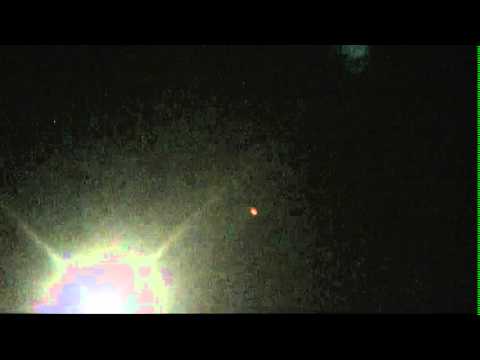The image depicts a dark, pixelated photograph with significant digital noise and widescreen black bars at the top and bottom. The background is completely black except for the lower left-hand corner, where a bright, multi-colored light radiates outward. The central core of the light is a bright white, surrounded by layers of pinkish tones, purples, blues, light reds, and bright yellows, creating a glowing aura around it. The light appears to be an intense headlight, possibly seen from inside a car at night, shining through a window. Additionally, there is a small green blob in the upper right-hand corner, and the entire image looks heavily compressed with visible digital artifacts, giving it a low-resolution, pixelated appearance.